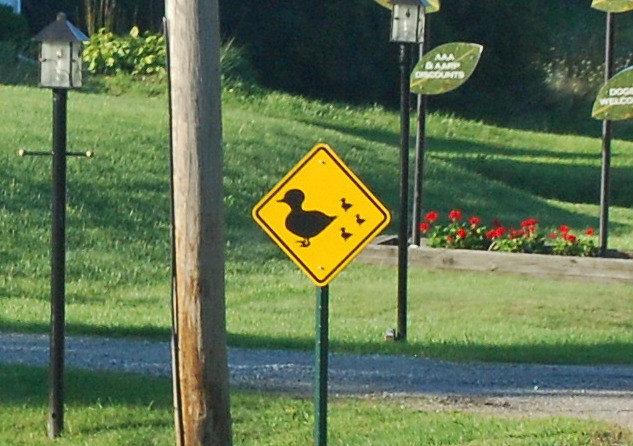In a serene park setting, green grass envelops the landscape, interspersed with rolling hills. A robust wooden electricity pole stands tall amidst the verdant scenery. Cutting across the bottom portion of the image, a neatly paved pathway stretches horizontally. In the foreground, a distinctively green pole anchored in the grass supports a yellow diamond-shaped sign. This sign features the silhouette of a mother duck leading her brood of baby chicks, signaling the presence of young ducklings likely indicative of spring. The sign serves as a gentle reminder for passersby to stay vigilant and protect these vulnerable creatures. The park exudes tranquility with its lush greenery and thoughtful signage aimed at preserving the local wildlife.